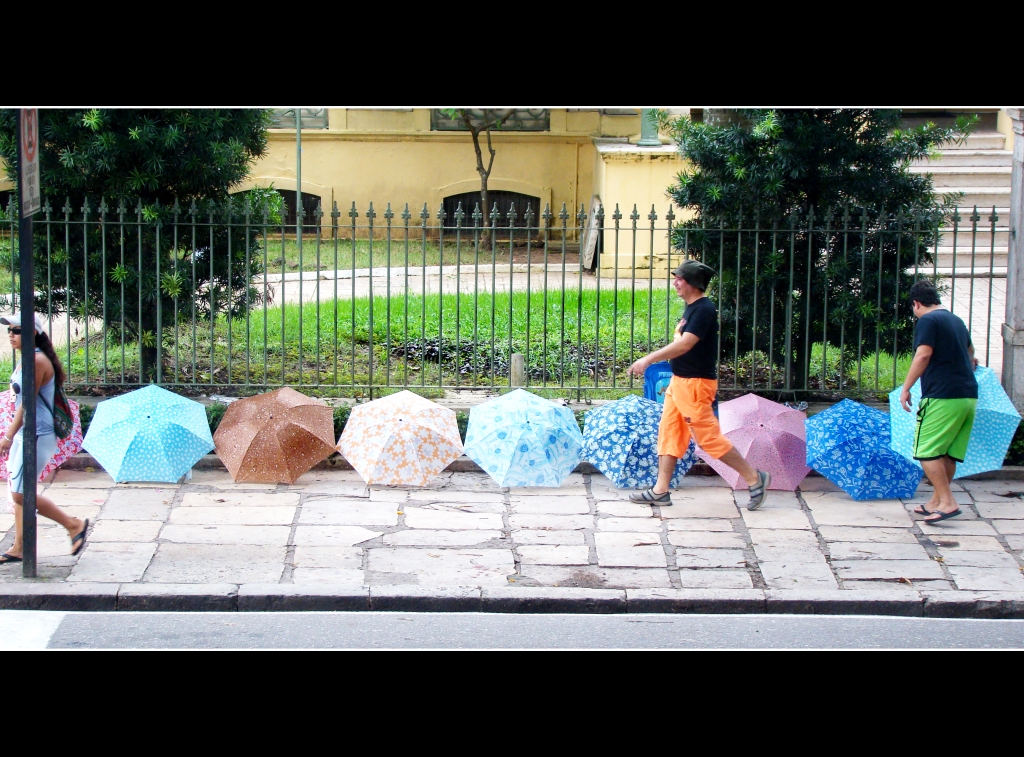The photograph captures an outdoor scene on a stone-paved sidewalk with large, rectilinear slabs. The focal point is a yellow building with an iron fence and two trees at the front. A series of colorful umbrellas, including blue, dark blue, light blue with a floral pattern, orange with white flowers, brown, and pink, are neatly laid out along the fence.

Three individuals are walking past the fence. On the left, a woman in sandals and shorts, carrying a backpack, and wearing a blue baseball cap and light sunglasses, strides towards the edge of the frame. To her right, two men, each in shorts—one in long orange shorts with a black t-shirt and a green hat, and the other in long green shorts, flip-flops, and a black t-shirt—accompany her. There is also a 'No Parking' sign facing the street. The building features steps leading up to a door and several windows, giving a hint of its potential residential or governmental use.